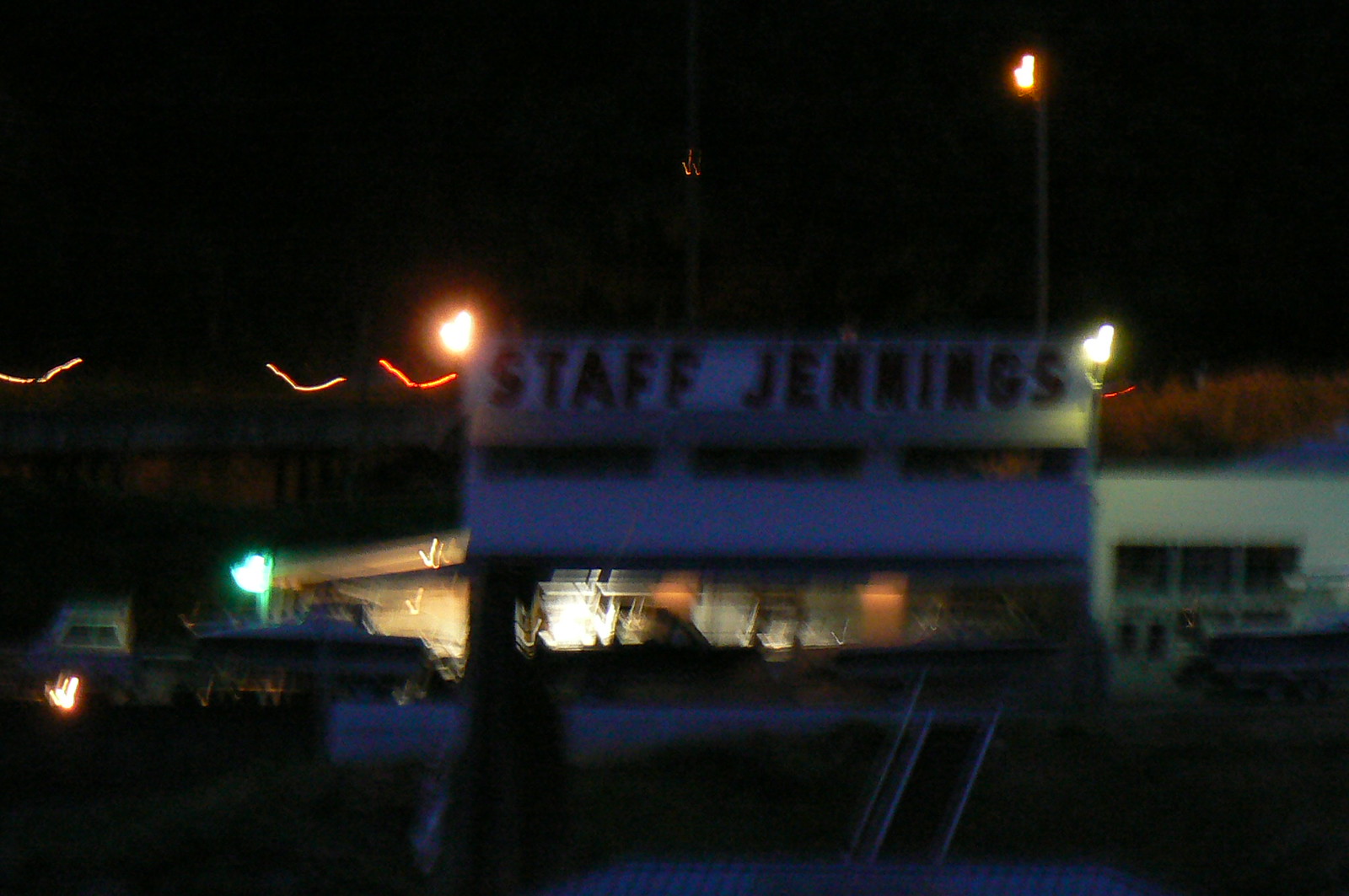The image depicts a nighttime outdoor scene with a black background. Central to the image, occupying the middle half, is an off-white, one-story concrete building that resembles a storefront. The building features a sign with red text that reads "Staff Jennings." Mounted on the upper corners of the sign are small lights, though they offer minimal illumination. The building, which has three square windows on its bottom right corner, is surrounded by several parked cars. In the distant background, additional streetlights and a building with illuminated windows can be seen, further enhancing the faint light in the scene. To the far left, there are two boats with distinct color patterns—a white-topped, blue-bottomed boat, and a white-topped, red-bottomed boat—adding to the marina-like atmosphere. The image quality appears grainy and slightly out of focus, especially around the periphery, contributing to its mysterious and subdued nighttime ambiance.